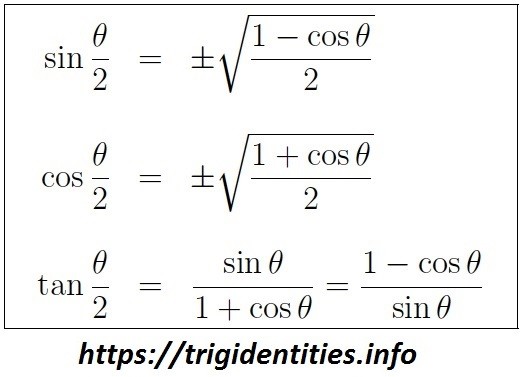The image displays a white box containing trigonometric identities, with the text in black. At the top of the box, the first equation reads: "sine of theta over 2 equals plus or minus the square root of 1 minus cosine of theta over 2." Directly below it, the second equation states: "cosine of theta over 2 equals plus or minus the square root of 1 plus cosine of theta over 2." The third equation, positioned underneath, is: "tangent of theta over 2 equals sine of theta over 1 plus cosine of theta, which also equals 1 minus cosine of theta over sine of theta." Beneath these equations, centered and in bold text, the website "HTTPS://trigidentities.info" is listed as the source of the information. The entire setup is formatted in a straightforward manner, suitable for referencing trigonometric identities.